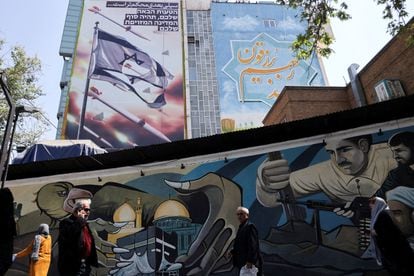The photograph captures a vibrant outdoor mural painted on the side of a building, set against a backdrop of bright blue skies and green trees. The mural in the foreground showcases a detailed scene with elements reminiscent of anime, featuring three figures, one of whom is intently working on a machine and appears to be holding a firearm or machine gun, all while dressed in a cream-yellow shirt. Adjacent to the scene is a man walking by, holding a mobile phone to his ear. 

In the background, the image reveals two towering glass buildings, each adorned with their own expansive murals. The building to the left displays what appears to be an Israeli flag with a Star of David set against a white background infused with hues of purple and dark tones. Conversely, the building on the right exhibits what seems to be Arabic writing accompanied by a star with more than six points, set against a backdrop that melds into the real blue sky and clouds. These overlapping layers of art and reality create a multi-dimensional, colorful, and lively urban scene.